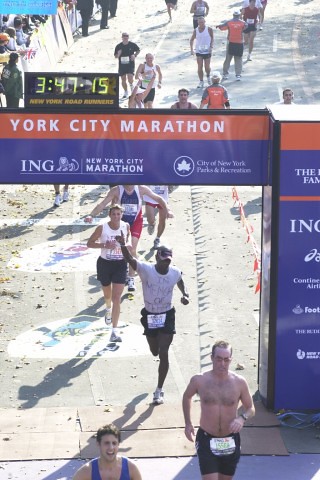The photograph captures the dynamic finish of the New York City Marathon with a diverse group of runners crossing under a blue and red archway emblazoned with the marathon's logos. Prominently displayed above the runners, a clock reads 3:47:15, marking their time. Runners, both male and female, many shirtless, briskly make their way through the arch in a lively action shot. At the center of the image, a man with dark brown skin, possibly African or African American, proudly raises his finger in a celebratory gesture as he passes directly beneath the archway. Behind him, other participants continue their efforts, and further in the background, security personnel and spectators, some jogging and some conversing, populate the scene. Visible signage includes a logo of the City of New York Parks and Recreation featuring a white maple leaf inside a white circle, and an ING logo with a lion. On the right side, a blue poster is visible, while spectators line the left side, cheering and observing the runners' final strides.